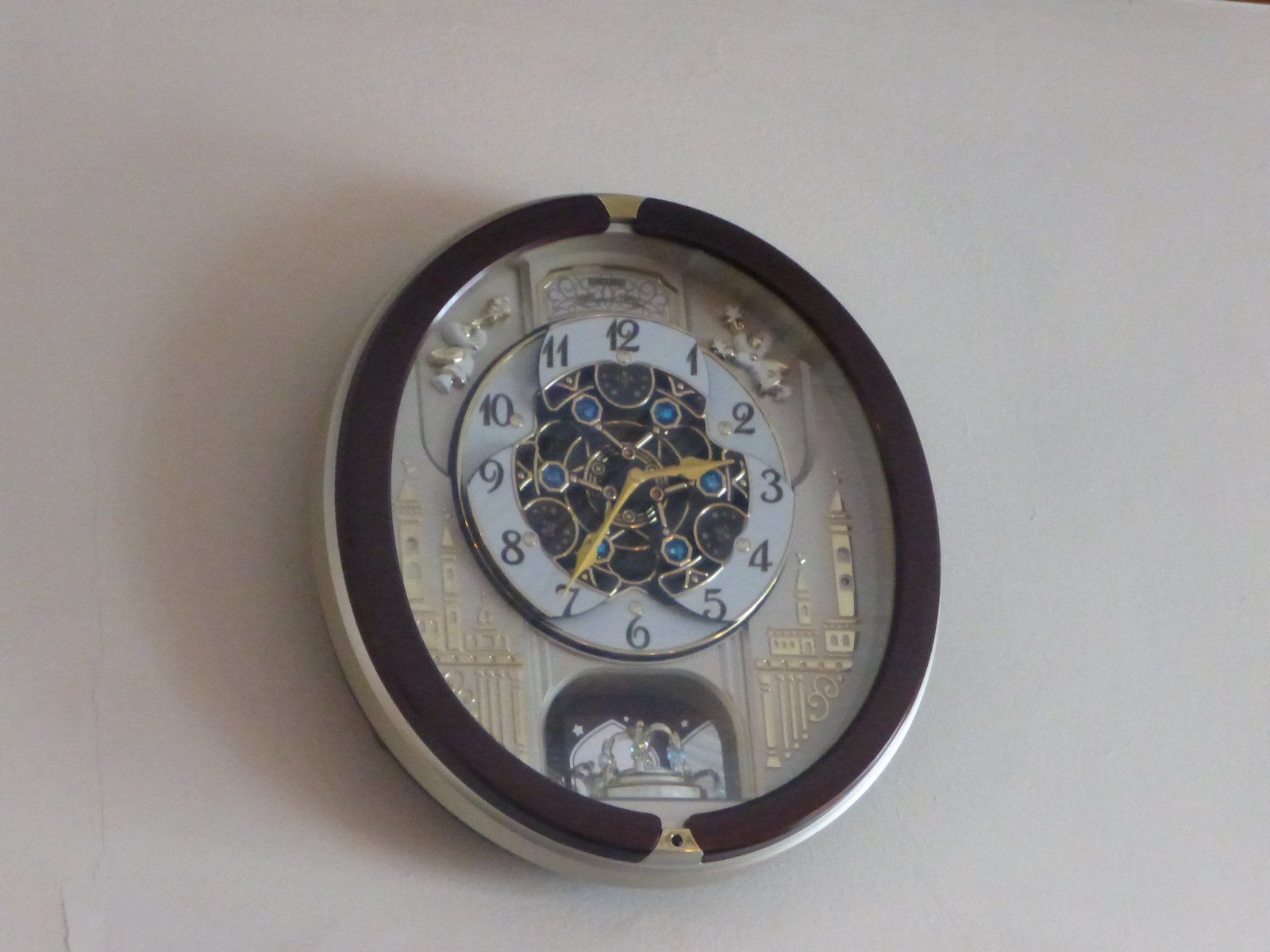A photograph depicting an extravagant egg-shaped clock hanging on a white wall. The clock features a darkish brown wooden frame with intricate gold accents. The face of the clock is predominantly black adorned with ornate gold designs and blue and red gemstone embellishments. The golden hands of the clock point to 2:35. Surrounding the face, which includes black, gold-outlined numerals, are elaborate details resembling a cityscape and possibly flowers, reflecting an Art Deco style. Below the clock face is an inset with more ornate decorations, including little angels playing trumpets and gold-outlined buildings, adding to its opulent appearance. The outer part of the clock is white, making the intricate interior stand out more vividly.